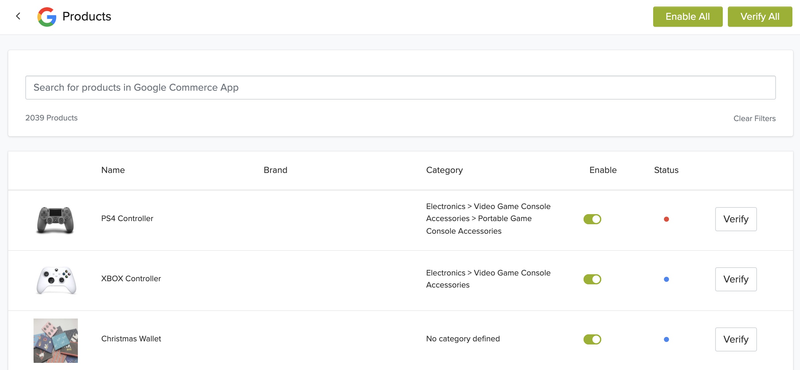The Google Commerce app's product verification interface displays 2039 products, including detailed status and categorization information. 

- First product: A PS4 controller, shown with a corresponding image. It falls under "Electronics," specifically "Video Game Console Accessories" and "Portable Game Console Accessories." The product status is "Enabled."
  
- Second product: An Xbox controller, accompanied by its image. This also belongs to the "Electronics" category and is listed under "Video Game Console Accessories." The status is "Enabled" and marked with a blue dot indicating verification.

- Third product: A Christmas wallet, depicted as a colorful array of squares featuring pink, blue, black, and white dots. This product currently has no defined category but is marked as "Enabled" and verified with a blue dot.

Additional functionalities include options to clear filters, search products by name, brand, or category, and verify or enable the status of individual items.